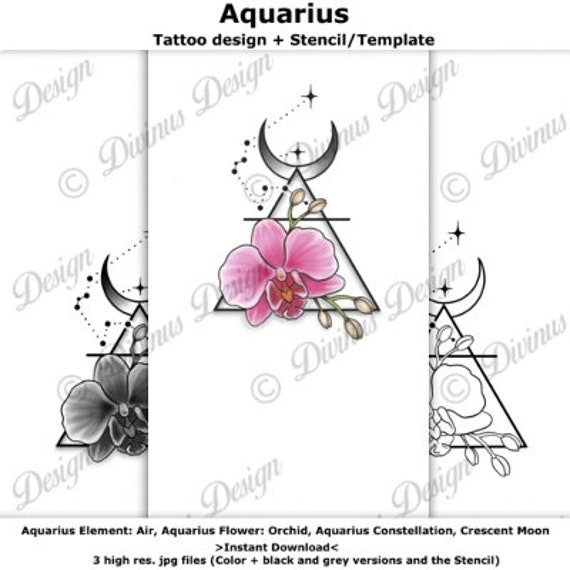The detailed image showcases a tattoo stencil centered around the zodiac sign Aquarius. At the top, "Aquarius" is prominently printed in black against a white background. Just below, the text reads "Tattoo Design plus Stencil/Template." Dominating the design is a triangle with an upward-turning crescent moon at the top, within which lies a vibrant purple-pink flower, likely an orchid, symbolizing the Aquarius flower. Flanking the central colored flower are two monochromatic variations: one completely filled in with black and gray tones, and the other just an outlined version. A watermark, reading "Divinus Design" with a copyright symbol in cursive, spans diagonally from the lower left to the upper right of the image, ensuring the design is protected. Beneath the main imagery, additional information is provided, including specifics about Aquarius: its element (air), associated flower (orchid), constellation, and crescent moon. The description also mentions the instant download availability, which includes three high-resolution .jpg files containing the colored, black-and-gray, and stencil versions of the tattoo design.